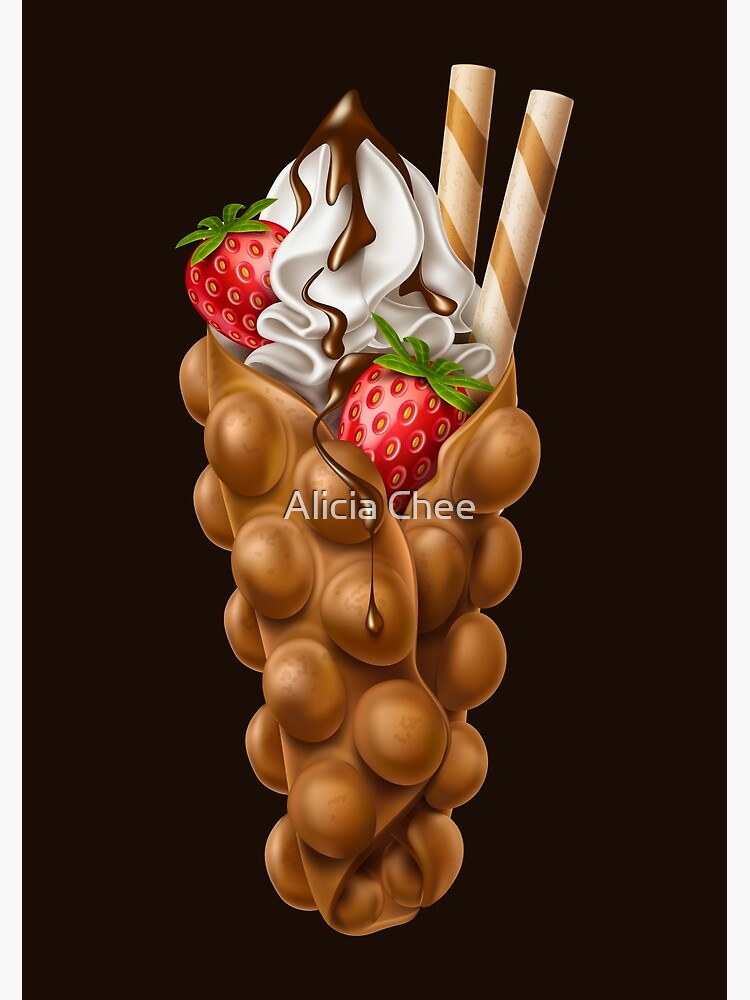This is a detailed digital illustration by Alice Chee, presenting a three-dimensional depiction of a decadent dessert against a stark black background. At the center of the composition is an intricate waffle cone, possibly made of chocolate and adorned with a nut-like texture, exhibiting a rich blend of brown and caramel hues. The cone is filled with luscious white whipped cream, which is generously topped with dark chocolate syrup that drips alluringly over the sides. Crowning the dessert are two vibrant red strawberries, complete with green stems and dotted with tiny yellow seeds, adding a fresh burst of color. Additionally, two striped straws, reminiscent of egg rolls with their whitish and light brown stripes, are positioned on the right side. The artwork is signed with the name "Alicia Chee" in white text, prominently displayed over the image, along with a transparent watermark.